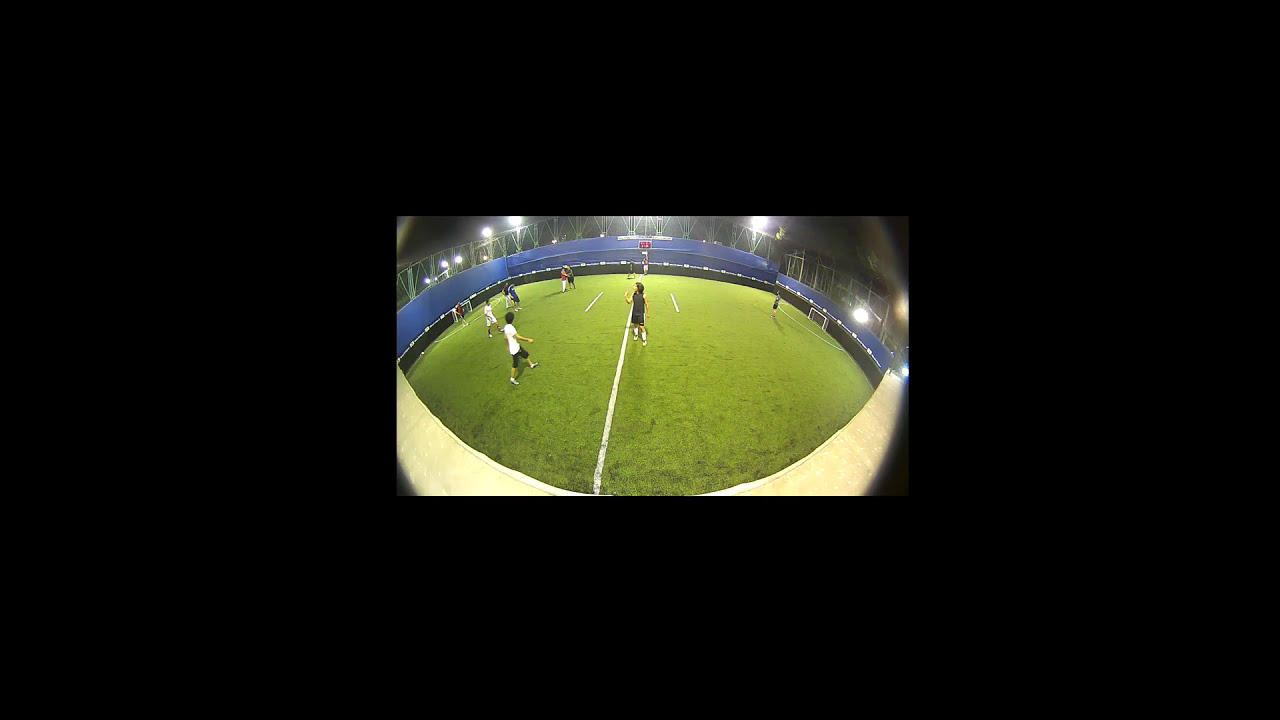The image features a heavily distorted photograph centered within a pure black background. The photograph, taken with a fisheye lens, displays an oval-shaped scene with extreme curvature, giving it a bulging appearance. Surrounding the field are dark barriers, padded in a mix of bright and navy blue. White distortions particularly mark the bottom corners of the image. Lit up by bright lights indicative of a nighttime setting, the small soccer field is lined with vivid green grass and marked with white lines, including curved lines in front of each goalpost situated on the left and right. Several young men, eight in total, are engaged in a casual or training game of soccer. The players wear varied attire: some donned in white t-shirts with dark pants, others in dark t-shirts, and one notably in a red shirt. The overall scene captures the dynamic energy of their game amidst the distinctive, warped visual effect.